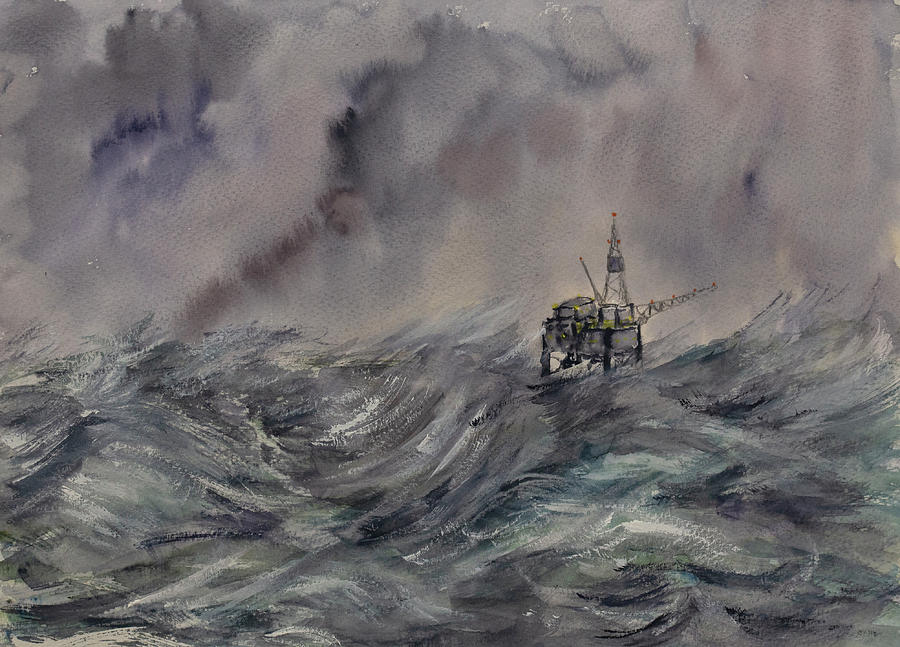The image depicts a detailed, hand-painted scene of an oil rig caught in the midst of a violent ocean storm. The rectangular painting, approximately six inches by four inches in size, appears to be executed with acrylic paints on canvas. It features a turbulent sea in the bottom half, characterized by dark, stormy waters rendered in various shades of gray, cream white, and a few streaks of black, blue, and green, highlighting the rough, tumultuous waves. Above, the sky is dominated by dark, swirling clouds painted in an array of grays and touches of red, along with purples and mauves, suggesting the severity of the storm. The oil rig sits just right of center, standing upright and painted predominantly in grays with accents of yellow on its body and small red lights on the radio tower and crane extending to the right. The fierce storm conditions are evident in the movement of the clouds and the agitated sea, capturing the oil rig's precarious position amid the chaos.